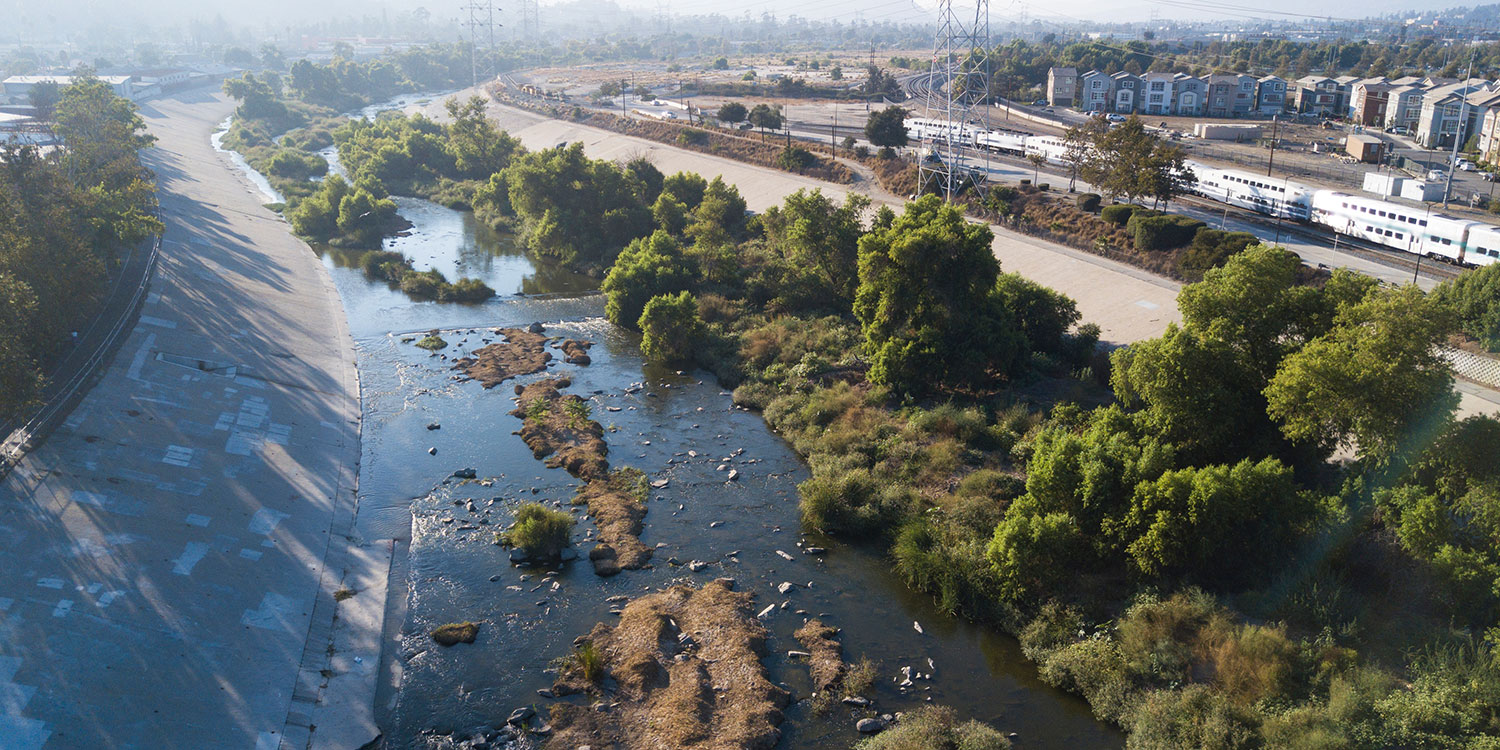This detailed panoramic aerial photograph captures a man-made river winding through a diverse landscape on a hazy sunny day. The river, appearing partially dried up with visible rocks at its bed, is flanked on the left by a sloped concrete retaining wall designed likely for flood control. In contrast, the right bank features a natural strip of ground dotted with shrubs and bushes. The elevated camera angle, approximately 30 feet above ground, reveals a richly vegetated area with a mix of vibrant green and brown trees, some of which extend into the shallow water littered with dirt and leaves. Adjacent to the river on the right, a road runs parallel to a parking lot area, leading to a curved semi-circle of residential buildings. In the distance, train tracks which pass by one side of the river stretch all the way to the horizon and merge into what appears to be a distant town or city.